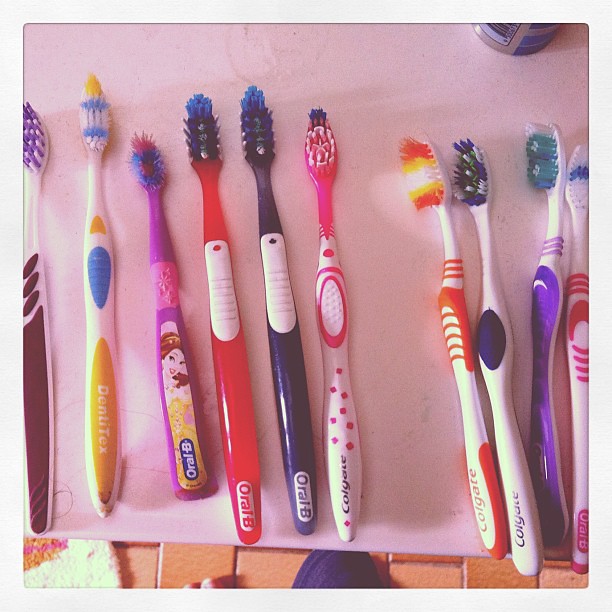The image depicts ten toothbrushes meticulously arranged in a row on a white counter, likely a bathroom vanity. Most of the toothbrushes are upright, with two slightly tilted to the side. The toothbrushes represent a variety of brands, including multiple from Dentex, Oral-B, and Colgate. A notable stand-out is a purple and pink children’s toothbrush featuring an image of Disney Princess Belle, indicating it's designed for kids. The toothbrush colors span a wide spectrum, with combinations including red and white, blue and white, pink and white, orange and white, yellow and blue, and purple and white. Each toothbrush has notably colorful bristles. In the upper right-hand corner of the image, partially cut off, is a bottle whose label and contents are not clearly visible. The white counter contrasts with an orange tile floor in the background, adding a warm, subtle detail to the scene.